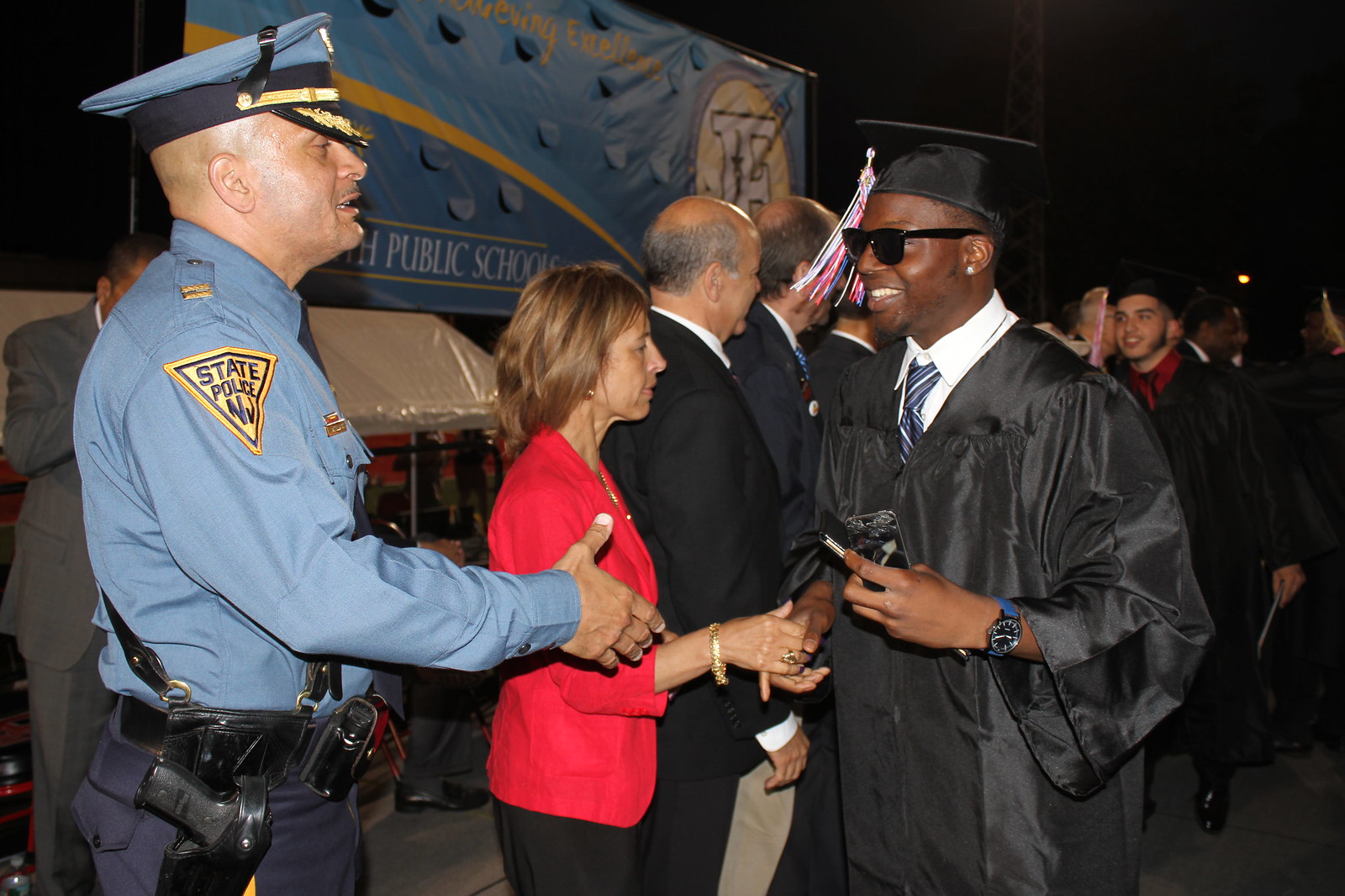In this image, we see an African-American male graduate with short hair and an earring, smiling as he participates in a graduation ceremony. He is wearing a black cap and gown over a white collared shirt paired with a blue tie. Notably, he has a blue watch on his left wrist and sunglasses. In his left hand, he holds a cell phone with a shattered screen and a padded diploma case, while his right hand is extended to shake hands. At the moment captured, he is shaking hands with a woman in a red jacket whose eyes are closed, and is poised to shake hands with a police officer in a blue uniform standing to his left. The ceremony is set on a stage draped with black curtains, and there's a blue banner in the background that reads "Public Schools," suggesting that this might be a high school graduation in Nevada. Other graduates in black gowns are lined up, also shaking hands with the attendees.